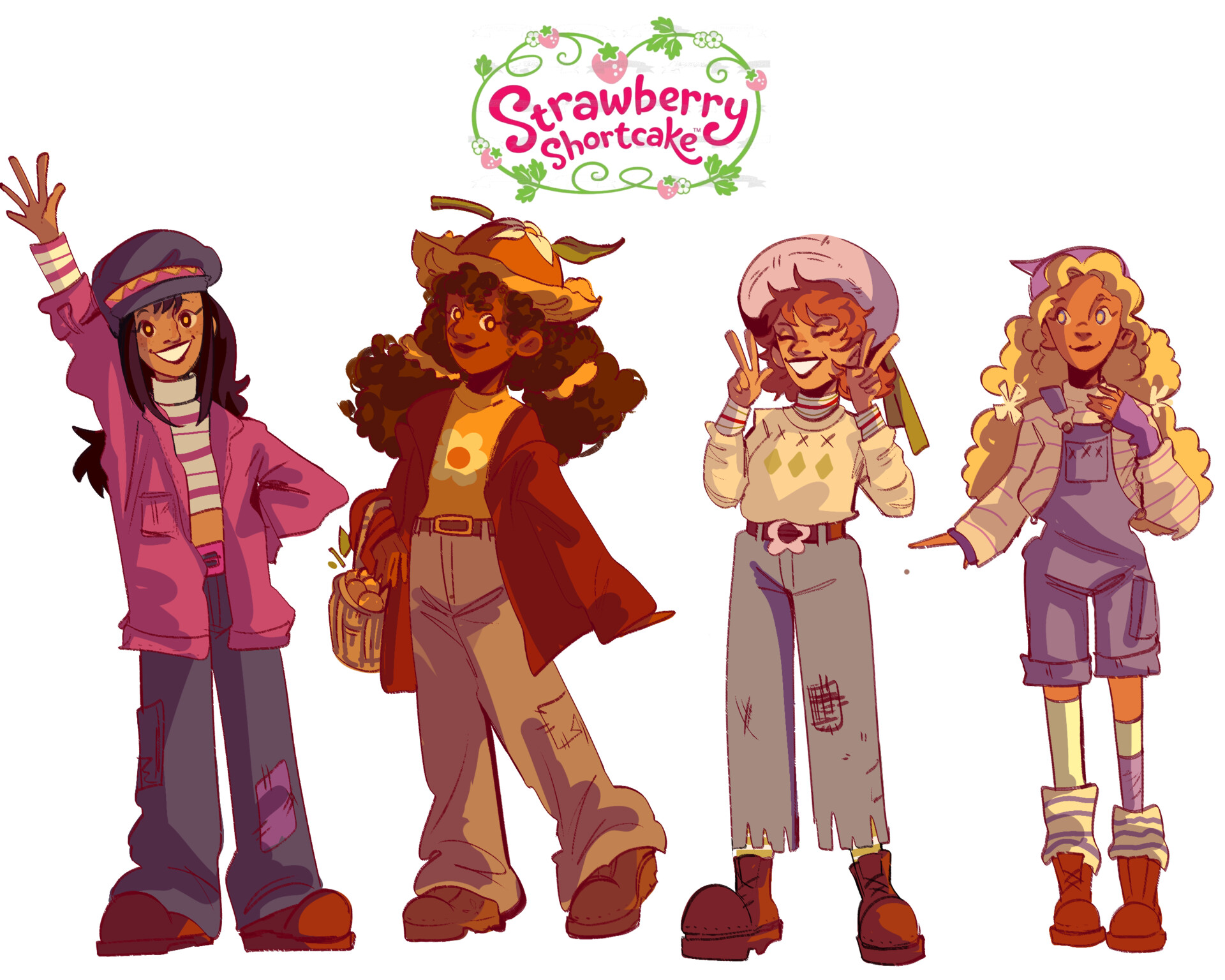This illustrated image features four trendy, teenage girl characters standing side by side, all appearing cheerful and stylish despite their seemingly lower-class attire. The text "Strawberry Shortcake" arches elegantly above them, designed as a logo with green vines adorned with pink strawberries and leaves. 

On the far left, a girl waves her hand with a smile, dressed in a pink jacket over a striped pink shirt, blue pants, and brown boots, completed with a navy beret. Next to her, there is a girl with curly brown hair and a smile, wearing a brown jacket, a yellow shirt with a white flower design, beige cargo pants, and dark brown shoes, while holding a basket and sporting a hat. 

Beside her, a girl with red hair styled in a distinctive manner is making a peace sign with both hands, dressed in a white sweater, blue jeans with a flower-buckled belt, and brown bulky boots, topped with a pink poofy hat. 

Lastly, on the far right stands a cheerful girl with long curly blonde hair, wearing blue overalls over a white striped shirt, long socks, and UGG-like bulky boots, finished with a pink hat. 

Together, they form a lively and vibrant group under the "Strawberry Shortcake" banner in this detailed and engaging illustration.